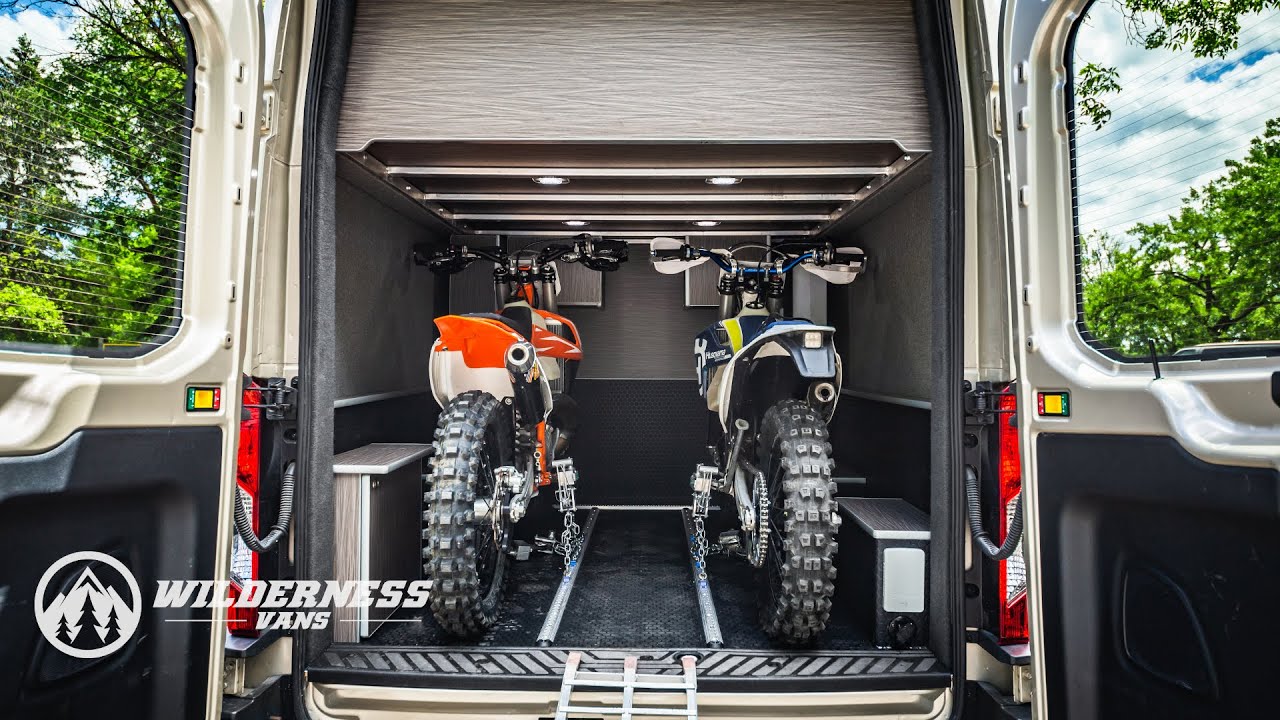This image features the open rear storage compartment of a van, branded as part of Wilderness Vans, as indicated by a logo and text in the bottom left corner depicting a mountain with trees. The scene captures a cloudy daytime sky and trees visible through the fully opened French-style rear doors of the van, suggesting an outdoor, possibly wilderness setting. Inside the van, there are two chained down motocross dirt bikes, the one on the left is orange and white, while the one on the right is black and yellow. The interior of the van is noteworthy, featuring a finished ceiling with inset overhead lighting that mimics a wood-like appearance. The floor is black, and small benches are visible on either side. The van’s storage area seems well-equipped, potentially for outdoor adventures, possibly with a ladder for loading and unloading the dirt bikes. Overall, this serves as a detailed advertisement highlighting the van's capacity to securely transport outdoor recreational vehicles.